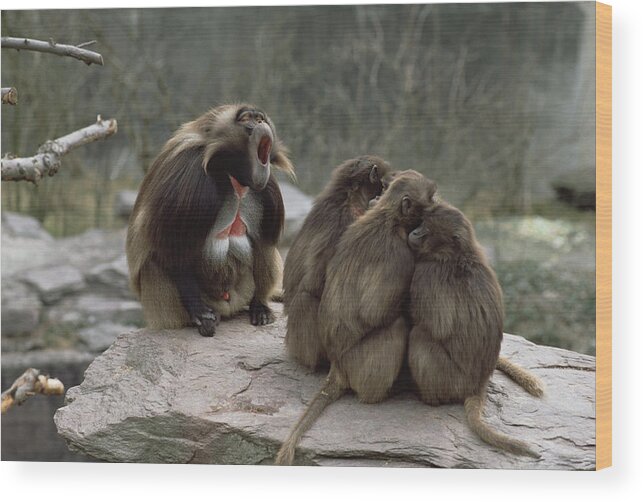In an outdoor setting with blurred brush and grass in the background, an image captures a group of baboons gathered on a large, flat, gray-tan rock. Three intertwined branches jut in from the left side of the frame. Central to the scene, three young baboons, tan in color, are huddled together with their tails extending outward. Their bodies are closely tucked in, exuding a sense of fear and vulnerability. A fourth baboon is partially visible in the background. Dominating the left side, a larger mother baboon, characterized by her tan and white fur with brown patches on her shoulders and arms, is in a striking pose with her mouth wide open, forming an oval shape as she appears to be screeching. Her prominent breasts add a notable detail. The overall composition, with its earthy tones of brown, tan, and gray, and the flat lighting, suggests that this photograph was taken outdoors during daylight, possibly in a natural or zoo setting.